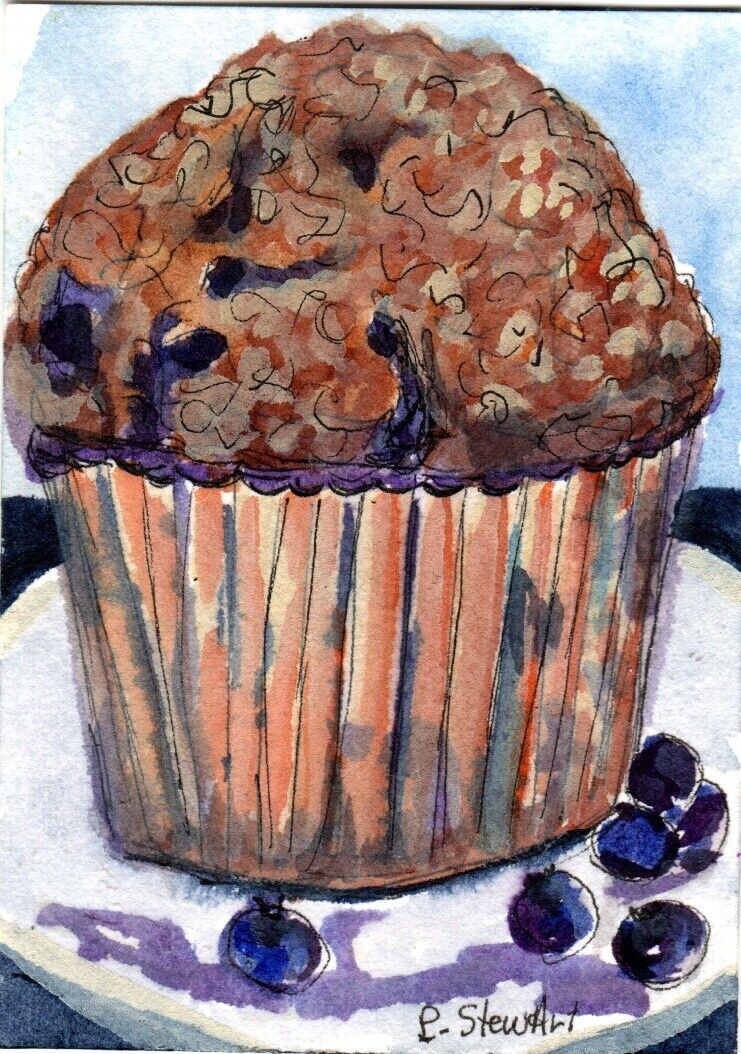The image features an abstract drawing likely created with markers, portraying what appears to be a blueberry muffin. The muffin, predominantly drawn in a non-realistic and abstract style, is placed within a light pink and orange muffin liner, speckled with blacks for added texture. The top of the muffin is depicted with crumbled brown hues, combined with purple spots symbolizing the blueberries. The top is further adorned with a tangle of black squiggly lines, enhancing the abstract theme. 

The muffin rests on a white plate, which showcases several blueberry spots. One prominent blueberry can be seen in the center, followed by a cluster of five more on the right side, alongside a representation of spilled blueberry sauce. The plate itself is distinctly circular. 

The background is filled with bluish watercolor strokes, serving as a backdrop and adding depth to the image without representing the sky.